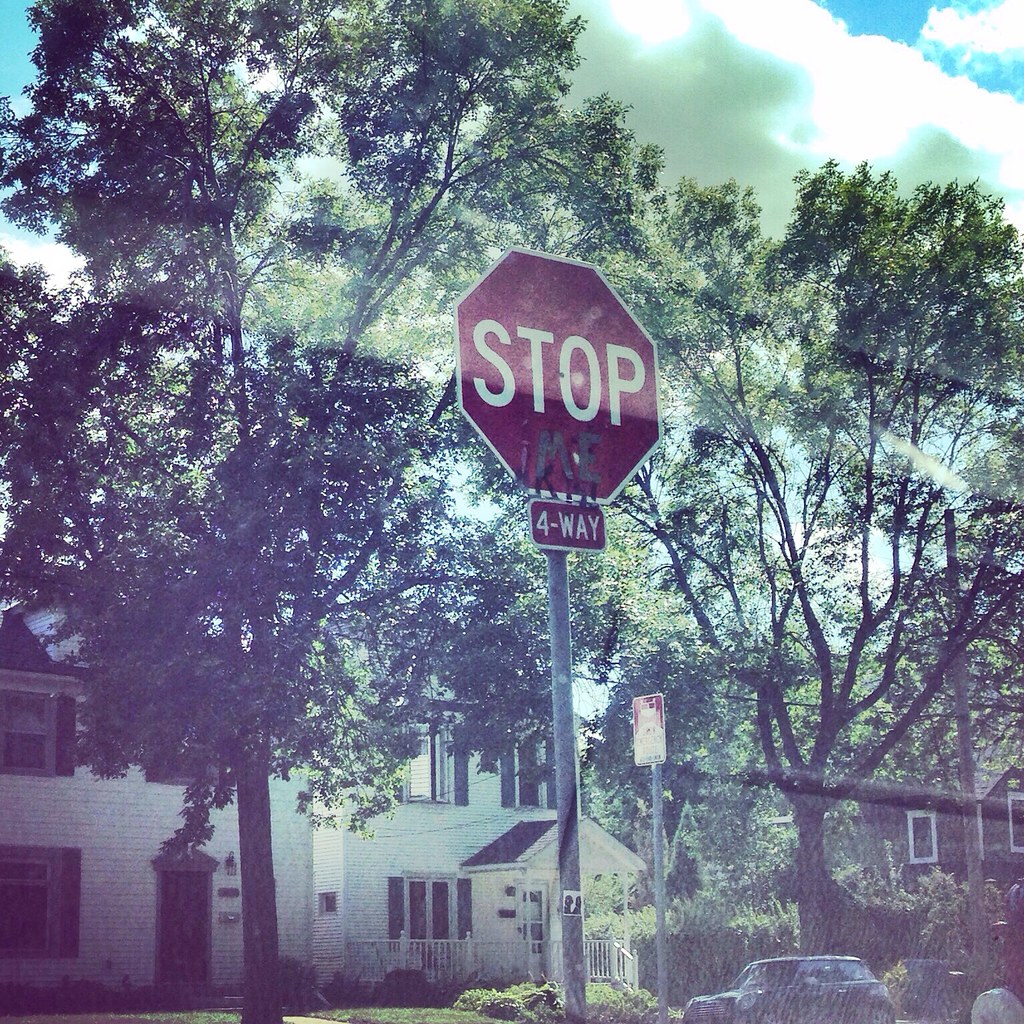Captured from the inside of a car, this photograph features a vivid red American stop sign prominently positioned against a picturesque residential backdrop. The sign, emblazoned with the white word "STOP," has been defaced with the graffiti "ME" in silver beneath the original text. Below the stop sign, a smaller sign indicates it is a four-way stop. Majestic green trees tower in the background, partially concealing rows of charming white houses. In the foreground to the right, a parked car is visible, while another darker-colored house is discernible in the distant right background. An additional, but unreadable, sign emerges faintly in the right part of the image, adding to the suburban scene's intricate details.